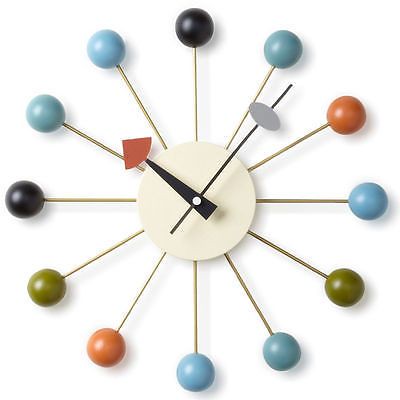The photograph features an abstract, analog wall clock set against a solid white background. The clock's central face is white, with two distinct hands: the hour hand is black with a red wedge at its tip, while the minute hand is also black but slimmer, ending in a gray circle. Extending from the clock's center are 12 golden rods, each tipped with a colorful sphere where the numbers would typically be. These spheres serve as the hour markers. Starting from 12 o'clock and moving clockwise, the colors are: black at 12, light blue at 1, red at 2, light blue at 3, green at 4, blue at 5, blue at 6, orange at 7, green at 8, black at 9, blue at 10, and blue at 11. The design creates a vibrant display with no numerical indicators, relying on the colored spheres for time-telling instead.